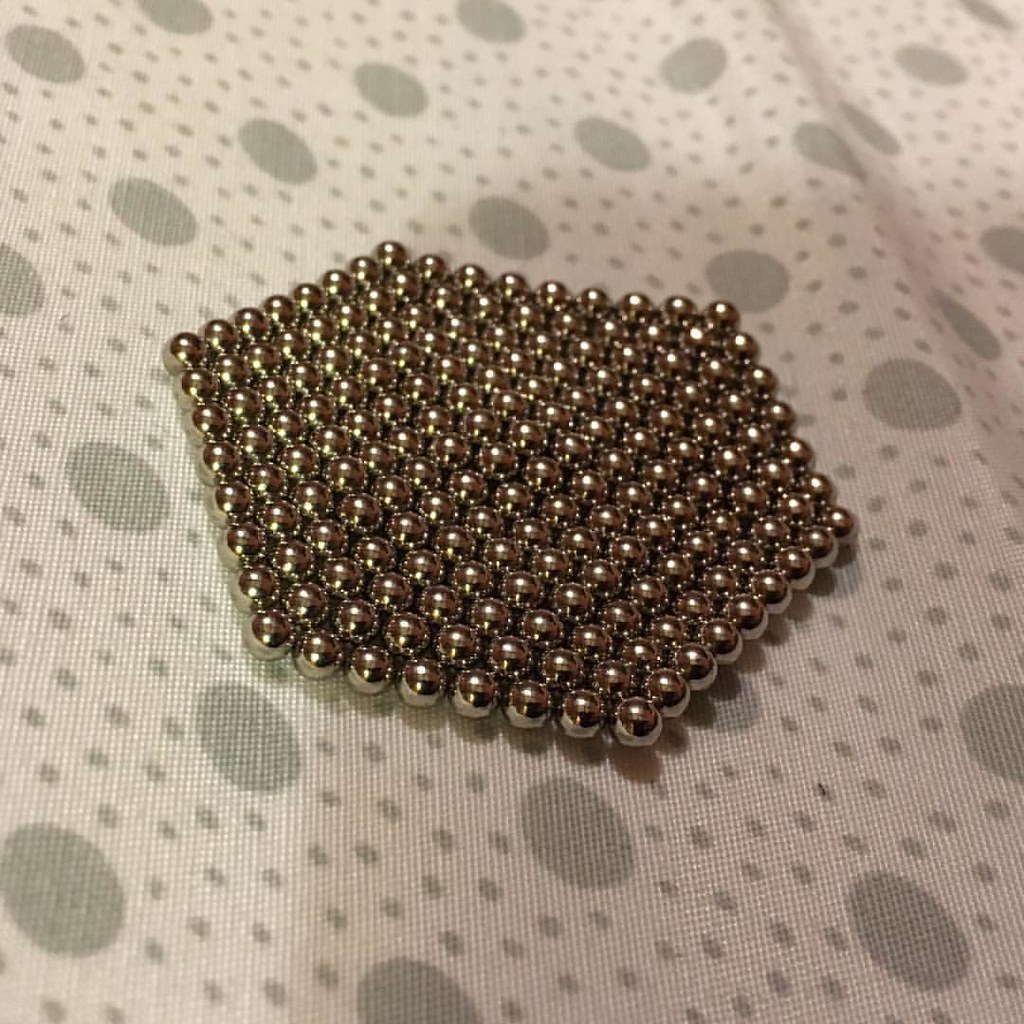The image features a densely packed hexagon of metallic, bright gold beads, perfectly aligned with no spaces between them. This hexagonal shape occupies the center of the picture, composed of layers of small beads intricately arranged to form the precise, six-sided figure. The beads are visually striking against a soft background that appears to be a textured material, such as cloth or a plastic mat. The background is beige adorned with a pattern of large, light brown or muted mint green circles and smaller polka dots of the same color, giving it a delicate, polka-dotted appearance. The image is a close-up, captured at an angle that reveals subtle creases in the material, enhancing the texture and depth of the background.